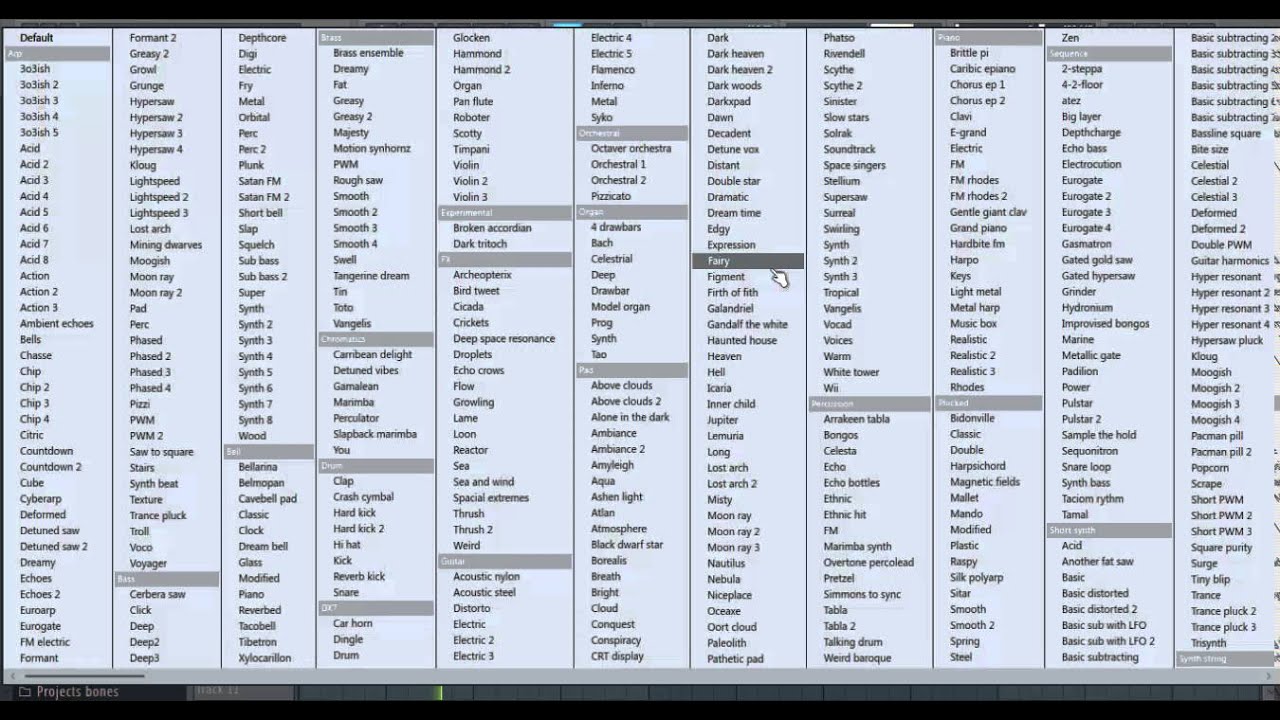This image features a detailed screenshot of a digital audio workstation (DAW) interface, showcasing an array of sound and instrument categories used for music production. The interface is primarily displayed on a clean, white background with small black text. On the far left, there is a column listing various categories, starting with 'Default' at the top, though the text beneath it is somewhat blurred and difficult to discern. 

Moving down the list, we observe clearly labeled categories that include 'Acid,' 'Bells,' 'Chip,' and 'Dreamy,' indicating various sound presets or types designed for different musical styles or effects. Further down, additional categories are organized alphabetically, such as 'Brass,' 'Bass,' 'Chromatics,' 'Drum,' 'Guitar,' 'FX' (presumably sound effects), 'Experimental,' 'Orchestral,' 'Organ,' 'Fairy' (possibly a whimsical or ethereal sound category), 'Percussion,' and 'Short Synth,' among others. Each category likely contains a range of specific sounds or instruments pertinent to the genre or style indicated.

Overall, this image captures a segment of a music production tool where users can select from a diverse palette of sounds and instruments to compose and produce music.